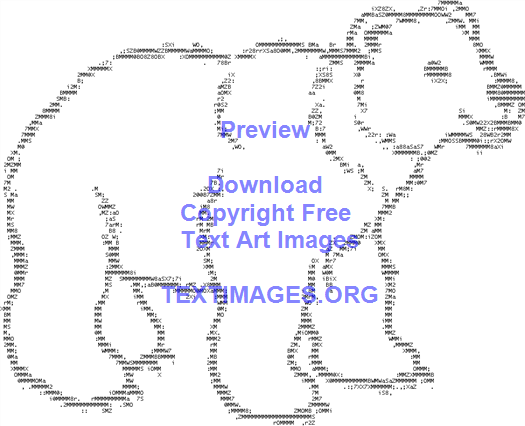This horizontal computer-generated image features an intricately detailed ASCII art drawing of a polar bear. The bear is composed entirely of staggered lines of text, arranged to convey a sense of curvature, texture, and depth. The bear's defining features include visible claws, a slightly open mouth, and distinct eyes and ears. Each part of the bear, from the eyes to the nose, is rendered using varying densities and boldness of letters and numbers, enhancing its lifelike appearance. 

The bear stands on all four legs, looking straight ahead with its head slightly raised. Superimposed over the center of the bear in purplish-blue text are the words "Preview," "Download Copyright Free Text Art Images," and "textimages.org," indicating the availability of free, copyright-free text art images from the mentioned website. This overlay reinforces the function of the image as a promotional visual for textimages.org, inviting viewers to explore and utilize the array of text art available there.